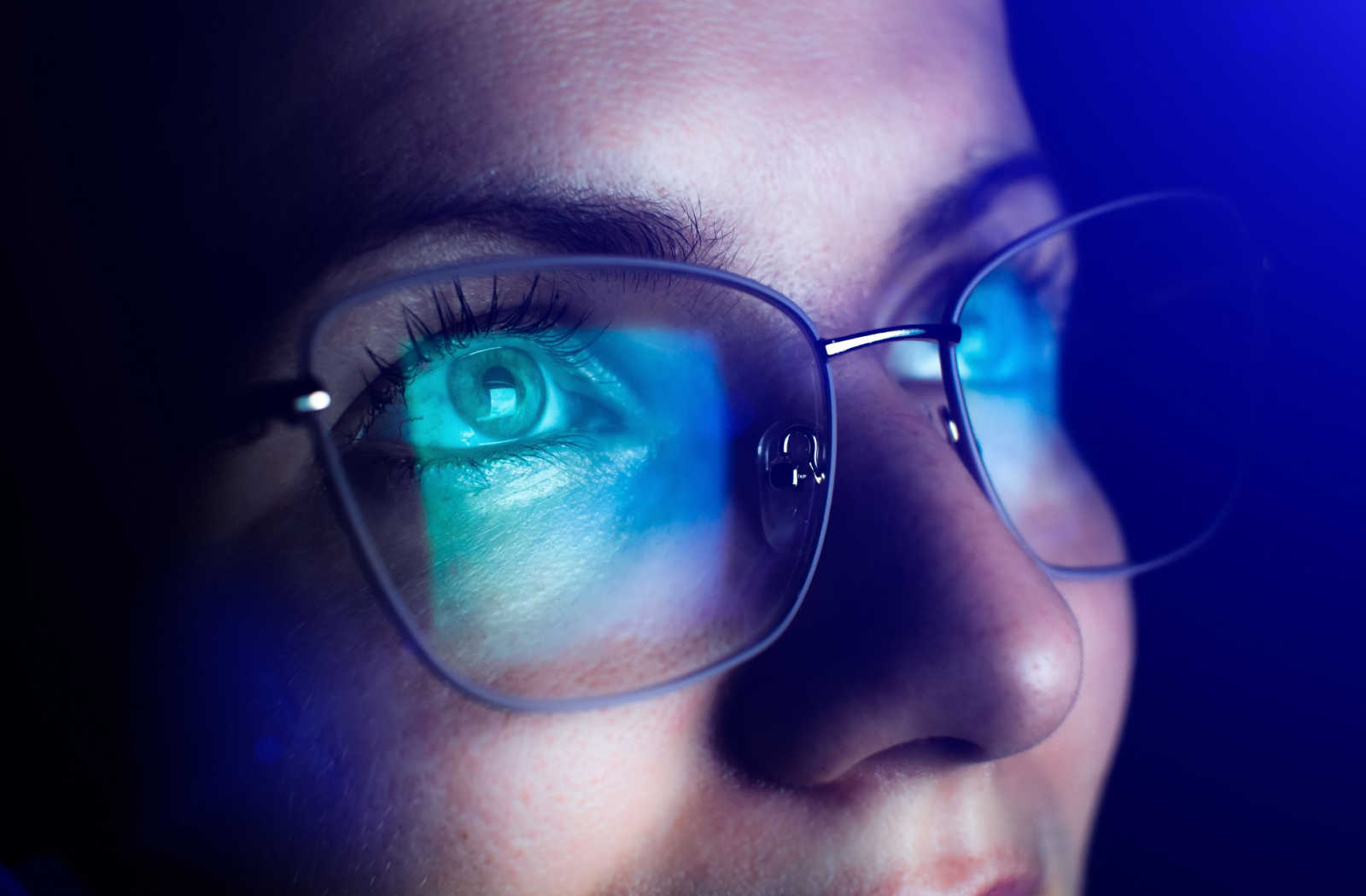This indoor photograph features a close-up of a white-skinned woman with green eyes, predominantly illuminated by the glow of a computer screen. She is wearing wireframe glasses with a metallic silver bridge and darker rims, possibly navy or black. The glasses have a rounded-off square shape reminiscent of 1950s designs. The computer screen's blue or teal light reflects prominently in her glasses, casting a blue tint on her cheeks and eyes. Her face is partially in shadow, especially around the nose and the left side of her forehead, while the rest is bathed in white light. The background is black, and the top right of the image has a subtle purple-blue hue. Only a portion of her face is visible—showing her eyes, nose, and the top of her lip—while her hair and ears remain obscured by darkness.